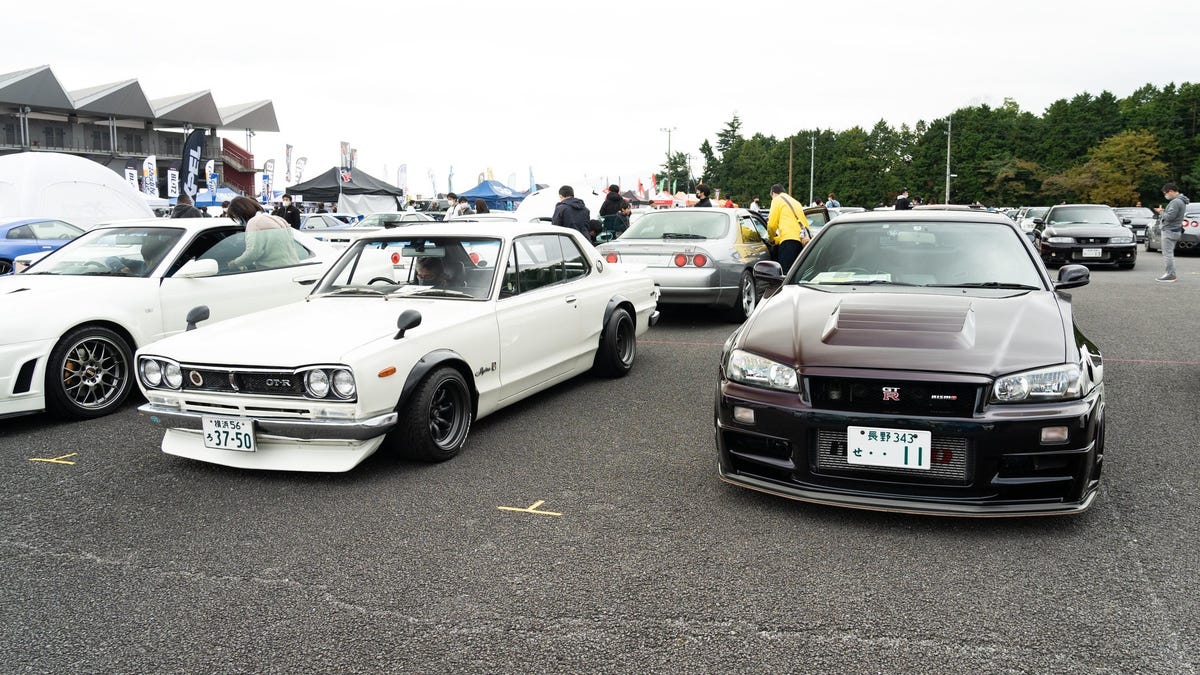The photograph captures a bustling scene at a car show in a parking lot, where various cars are meticulously parked in rows stretching from the left to the right of the image. A notable variety of cars are displayed, including a distinctive white Camaro in the left-middle section, a vintage sporty white car from the 60s or 70s, and a brown car, alongside a mix of white, silver, and black cars. Attendees are seen mingling around the vehicles, adding to the lively atmosphere. In the background, the upper right corner features lush green trees, while the upper left showcases a striking, modern-style building with four peaked roof sections. The sky is white, suggesting a mid-day setting. The scene notably blends the excitement of a car show with the structured layout of a parking lot, evoking a sense of community and shared enthusiasm for automobiles.